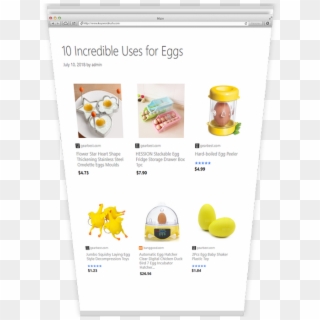The image depicts a detailed view of a webpage against a checkerboard background in light gray and white. At the top, it features a typical web browser interface, including an address bar and a search bar. Adjacent to these bars are a set of colored dots—yellow, green, red, yellow, and green—aligned horizontally.

Below the header, the main content of the webpage is displayed on a white background with gray text. The headline reads "Ten Incredible Uses for Eggs." Below this headline, there are six images arranged in two rows.

In the first row of images:
1. The left image shows eggs poured into cookie cutters and cooked, appearing sunny side up.
2. The middle image is unclear and indistinct.
3. The right image depicts an egg inside a plastic container.

In the second row of images:
1. The left image is obscure and challenging to interpret.
2. The middle image shows egg yolks seemingly formed to resemble small chickens.
3. The right image displays an egg inside a plastic dome with a green and yellow base.

Each image has accompanying text below it, which also includes prices; however, the text is too small to be legible.